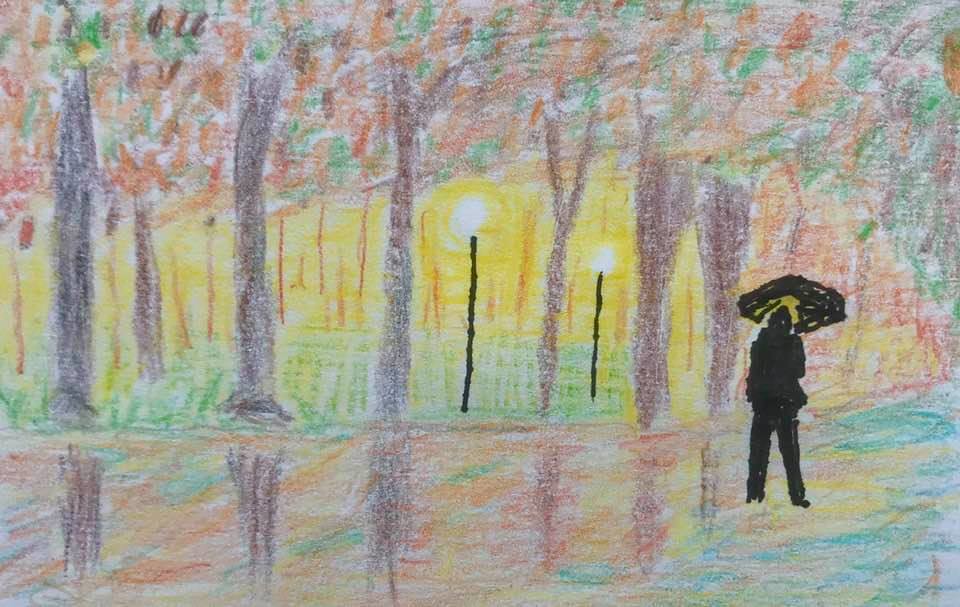This detailed mixed media painting, possibly created with crayons and colored pencils, depicts an autumnal scene centered around a solitary black silhouetted figure holding an umbrella at the far right. The background features a dense array of trees with a harmony of orange, green, and brown leaves intertwined, stretching from the left to the right. The trees, which have purplish-brown trunks, frame the scene and extends upward to create a vibrant canopy of autumn foliage. In the middle of the composition, there are two black streetlights with circular fixtures casting a bright yellow glow, illuminating the area. The yellow light blends into the background, creating a warm ambiance. The ground beneath the trees and the figure is glossy, suggesting it is wet, as evidenced by the reflection of the trees, spanning from the left to the right. The scene captures the essence of a rainy fall evening, with intricate details in the textures and colors used, making the mixed media approach evident. The expansive image, wider than it is tall, does not contain any visible artist signature.